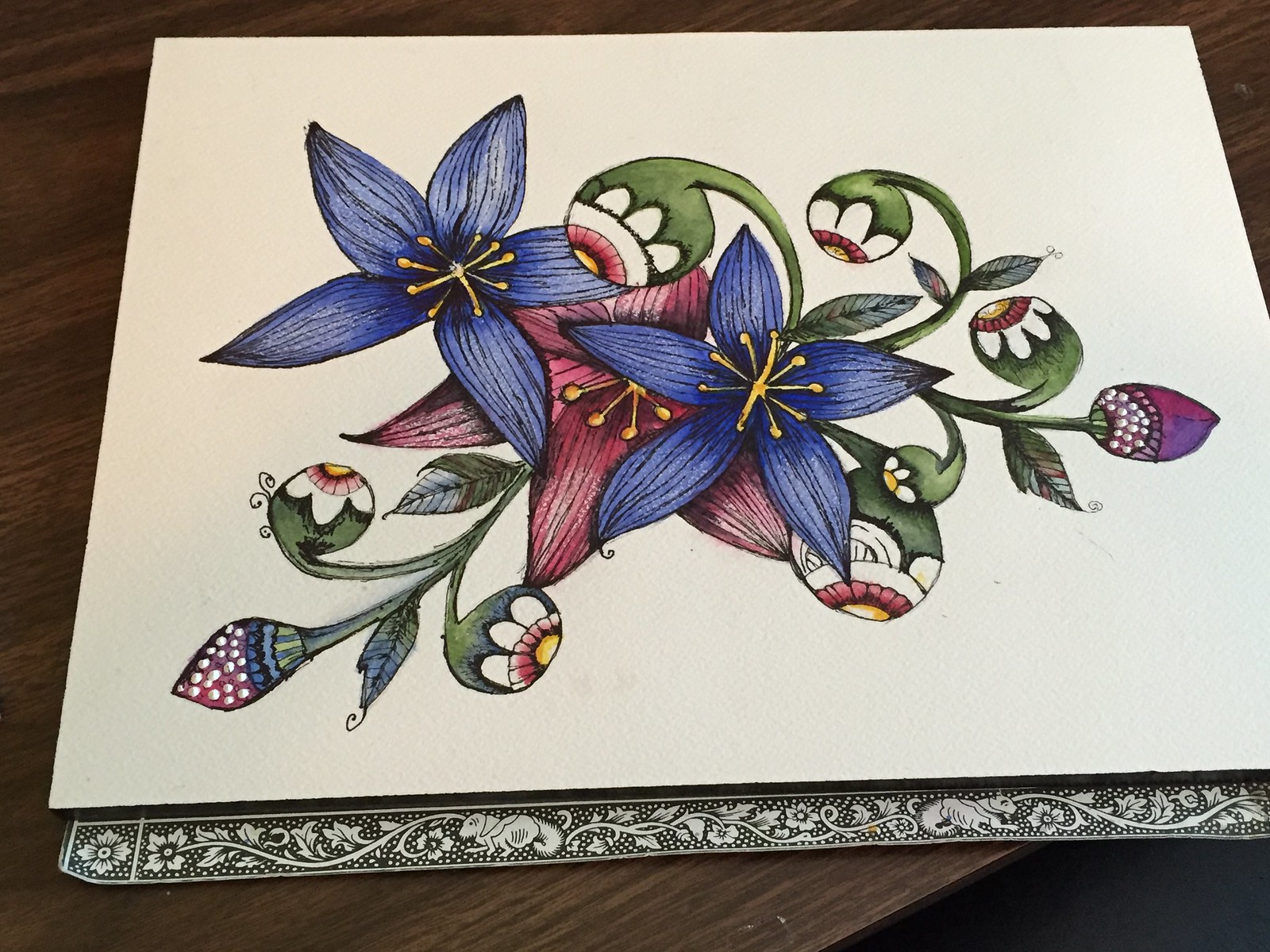This image features a highly detailed piece of artwork, most likely a painting, displayed on a thick piece of white board with an elegant ribbon border along the bottom. The composition centers around various intricately rendered flowers. Dominating the scene are large royal blue flowers with gold tendrils in the middle and dark dusty rose-colored flowers, also featuring gold tendrils. In the background, a pink flower with a golden center adds a splash of contrast. Green stems wind through the piece, leading to green bulbs tipped with white petals and surrounded by what appear to be small, eye-like designs with yellow centers and red borders. Several flower buds in hues of dark red or purpley-red, resembling closed rosebuds with tiny pearls beneath them, are interspersed throughout the painting. Set against a dark wooden tabletop, a sketch pad is partially visible, featuring tabbed pages adorned with black-and-white illustrations of flowers and rabbits. This scene captures an artist’s meticulous work with markers, detailed down to the flower buds, highlighting a rich tapestry of colors and botanical beauty.